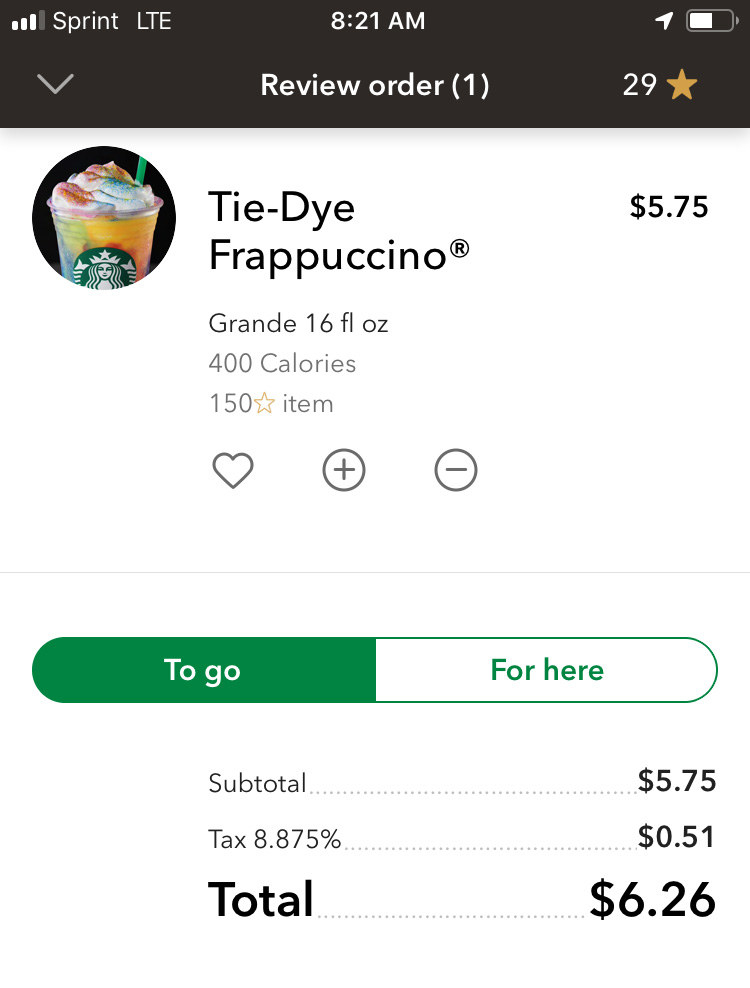A mobile screenshot displays an order screen for a colorful Tie-Dye Frappuccino from Starbucks. The drink, captured vividly in yellow, blue, and red hues, is housed in a clear plastic cup emblazoned with the iconic green and white Starbucks logo, showcasing half of the siren with flowing hair. The background behind the Frappuccino image is stark black. 

Above the order details, the phone runs on Sprint with an LTE connection, indicated by small icons at the top. The customer has reviewed their order, marked as "1" in line with an accompanying star symbol, time-stamped at 8:21 a.m. The item ordered is a Grande (16 ounces) Tie-Dye Frappuccino, costing $5.75 and totaling 400 calories, also providing 150 reward stars. The drink is for takeaway, as denoted by the “to-go” option. 

The subtotal of the order is $5.75, with an added tax of 8.875% amounting to approximately 51 cents. The final total stands at $6.26. The display features a predominantly white background, except for the upper section showing the phone's status information set against a black backdrop.